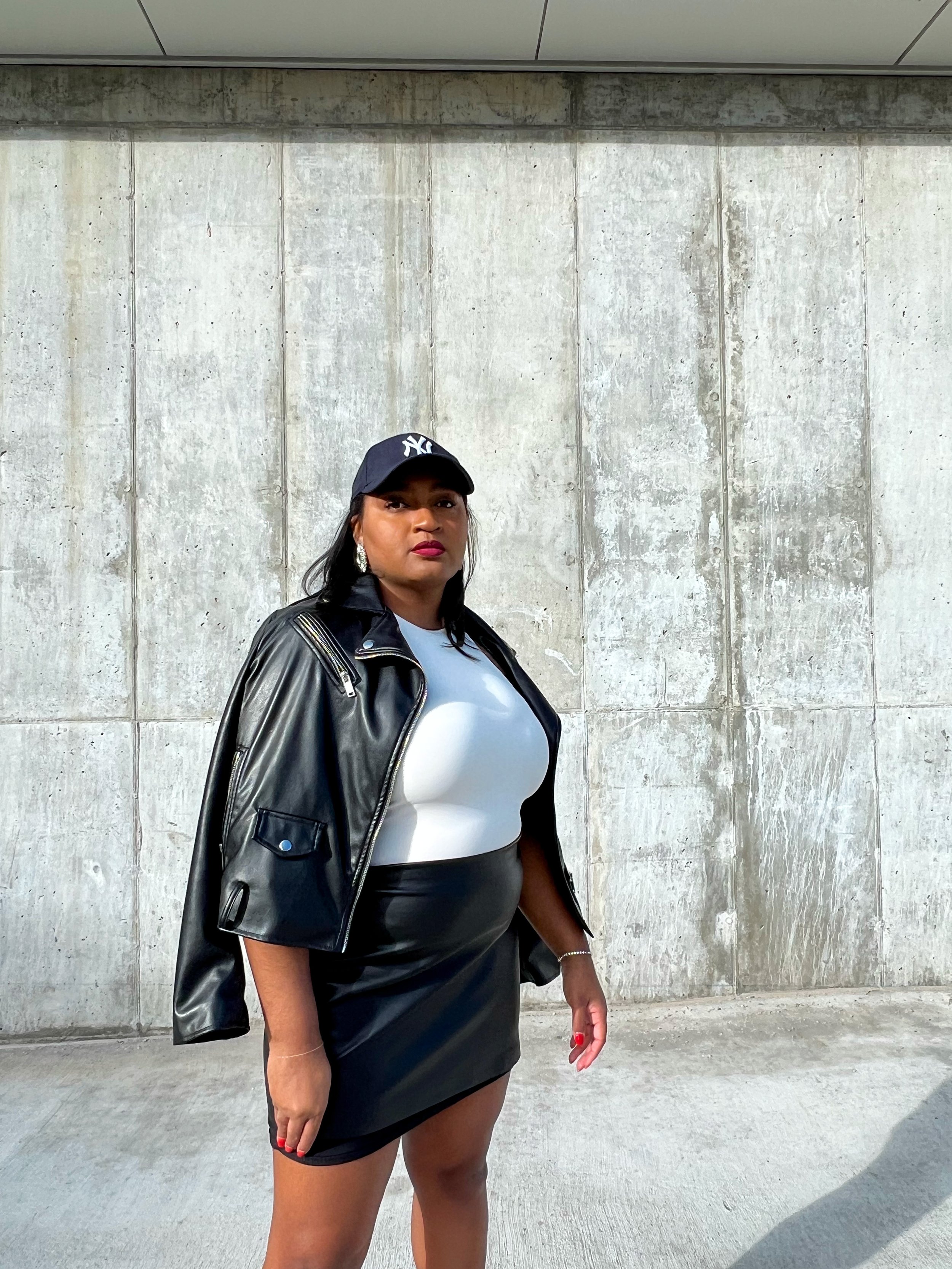In this striking fashion-forward photo, an African-American woman stands confidently against a stark, minimalist backdrop of plain concrete. The photo is brightly lit, emphasizing the sharp contrast between her bold outfit and the subdued environment. She's wearing a dark blue New York Yankees ball cap, hoop earrings, and striking red lipstick, all of which highlight her poised look. Her attire features a fitted white t-shirt tucked into a black leather or pleather miniskirt, paired with a matching black leather or pleather crop jacket draped over her shoulders. Accentuating her look, she wears a silver bracelet on one wrist and her fingernails are painted red. The concrete ground beneath her and the wall behind her enhance the photograph’s clean and modern aesthetic, focusing all attention on her chic ensemble.